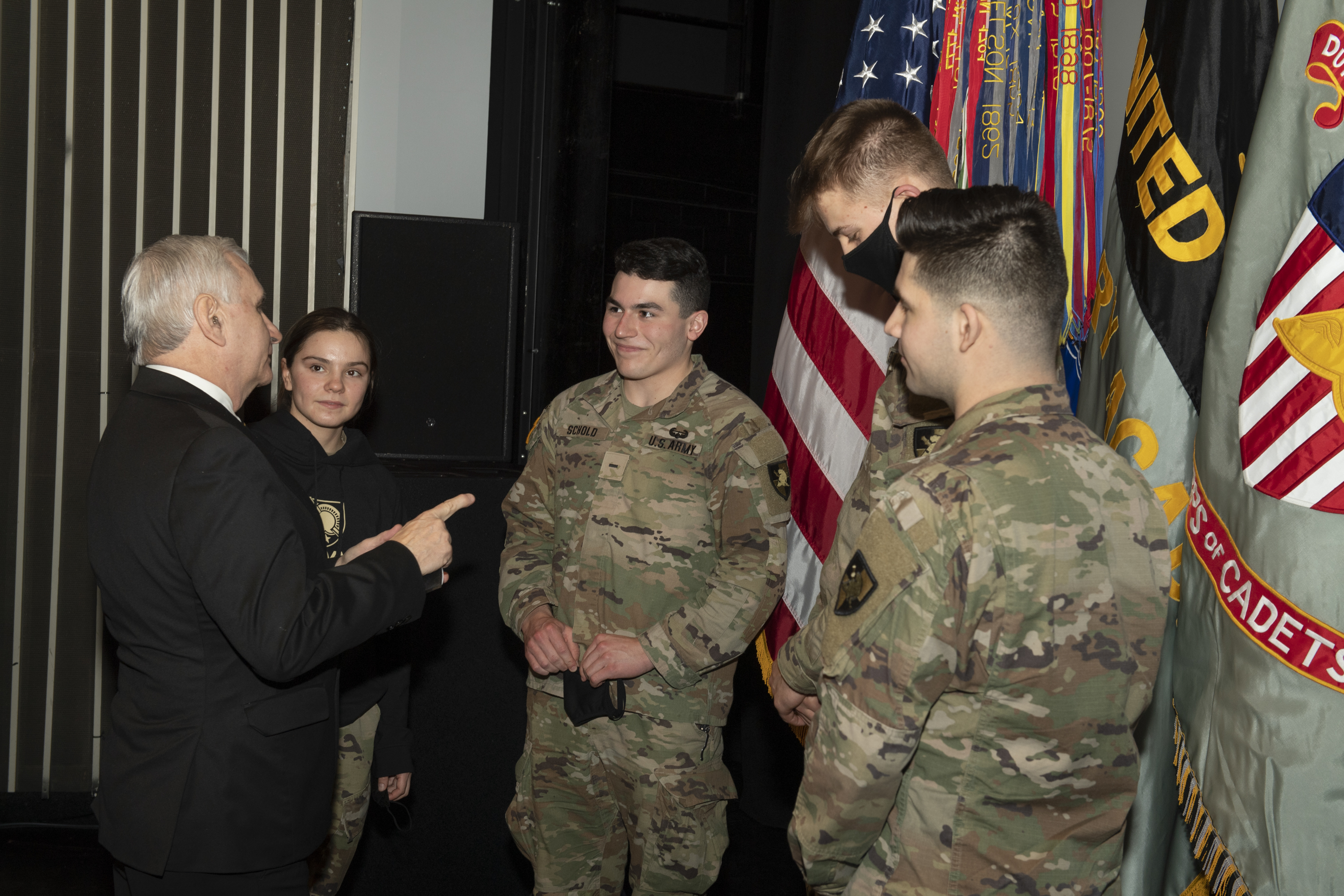The photograph captures an indoor ceremony or event featuring four young U.S. Army soldiers, three men and one woman, speaking with an older man. The man, dressed in a black suit and sporting gray hair, is on the left side of the image, mid-speech, and pointing towards the soldiers. The soldiers, appearing to be in their late teens or early twenties, are dressed in standard camouflage uniforms, though the woman is also wearing a black hoodie underneath her camo jacket. One of the soldiers is also seen wearing a dark COVID mask. They are standing against a backdrop of several flags; prominently visible are the American flag and another with the word "United" in yellow on a black field. The scene is set against a dark background with additional colorful ribbons and stripes from the flags adding contrast. The soldiers are attentively listening to the man, creating a moment of interaction and engagement.